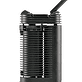The image features a predominantly black, cylindrical object set against a stark white background, occupying the center of the frame. The item has a spout or short straw protruding from the upper right corner. The cylinder's side displays horizontal grooves, revealing a solid black interior behind them. Near the object's base is some text, potentially depicting a brand name starting with the letter "C," although it is partially obscured and difficult to read. Adjacent to this text is a small, illuminated green light. Additionally, there are orange mechanisms or buttons on both the left and right sides of the object, with the right one being slightly larger. Sporadically, there are also three small blue areas visible on the object. The object appears to have functional aspects, such as vented slits and raised ridges, suggesting it might be a tool, space heater, or an unconventional drink container.